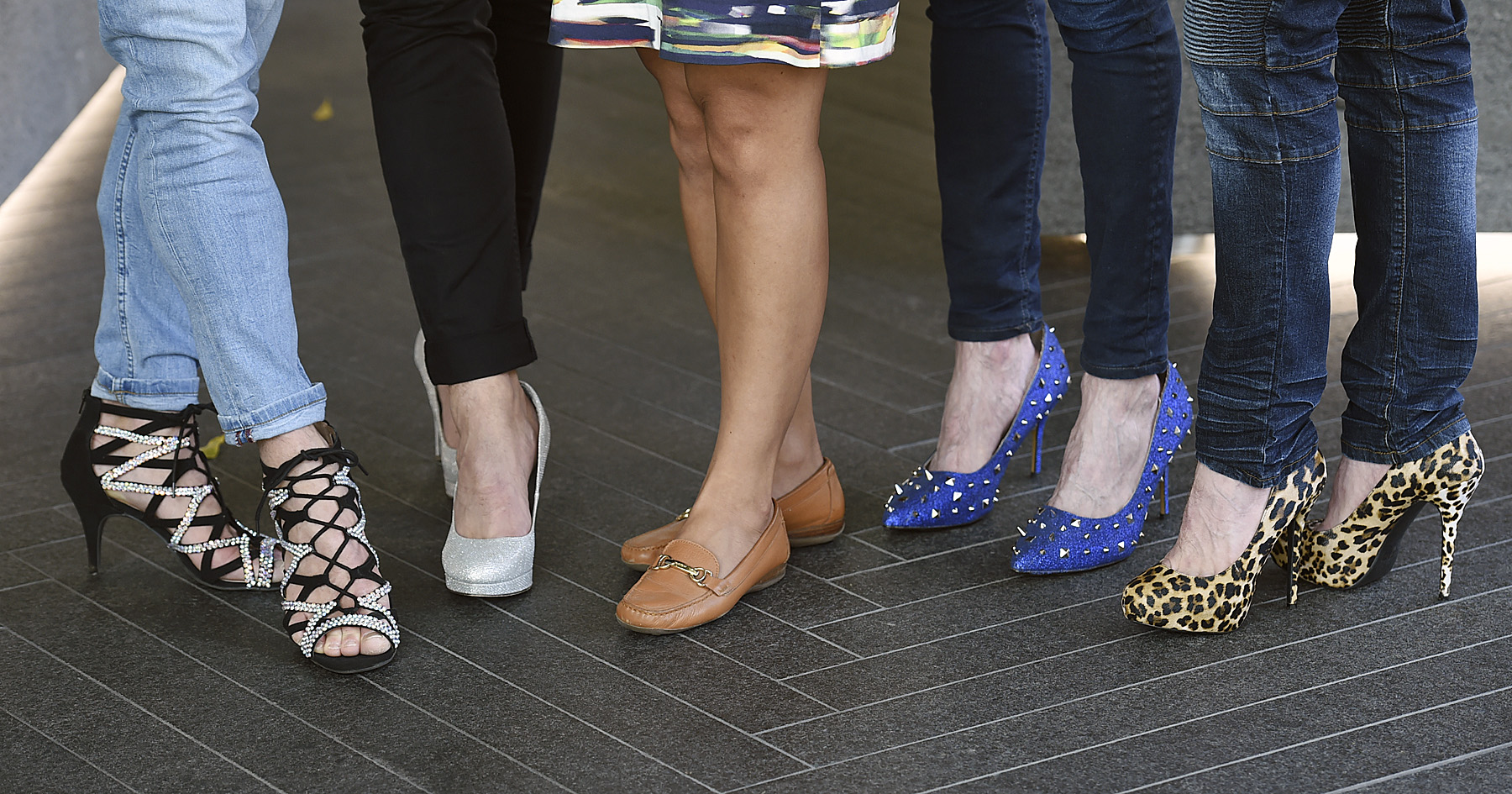The photograph showcases the lower legs and feet of five women, all with fair to light skin tones, standing on a dark gray, herringbone-patterned stone tile floor. From left to right, the footwear and attire are as follows:

- The far-left individual is wearing blue jeans paired with black high heels adorned with white and diamond-like open-toed straps.
- Next, a person in long black pants is wearing off-white high heels, facing the viewer.
- The middle figure, who has slightly darker skin, is in a colored skirt, sporting brown flat shoes with a gold buckle at the front.
- To the right, one person is wearing dark blue jeans with blue high heel shoes accentuated by gold metal spikes.
- The far-right individual wears dark blue jeans and leopard-patterned high heels.

The background includes a gray stone wall and a white underlight illuminating the pathway, adding a modern touch to the scene.